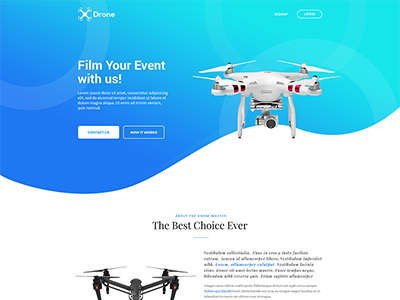The image depicts a web page for a company named "Drone" that promotes drone-related services. The top section of the page features a header with a gradient background transitioning from bluish tones to a light teal. The header includes the company logo, which incorporates an image of a drone to the left of the text.

Below the header, a prominent banner showcases two drones. The top drone is white, equipped with four propellers and a camera, emphasizing its role in aerial photography or videography. Accompanying the drone image is the tagline "Film your event with us!" and a caption declaring "The best choice ever." However, there are two buttons near this area that are too blurry to read clearly.

In the section below, a black drone is displayed, mirroring the design of the white drone with four propellers. The positioning of the propellers suggests that each drone has one propeller at the end of each of its four arms, although the direct frontal perspective makes it difficult to ascertain the exact configuration.

Overall, the web page blends a professional layout with strategic use of color contrasts to highlight its services and the technology offered by the company "Drone."